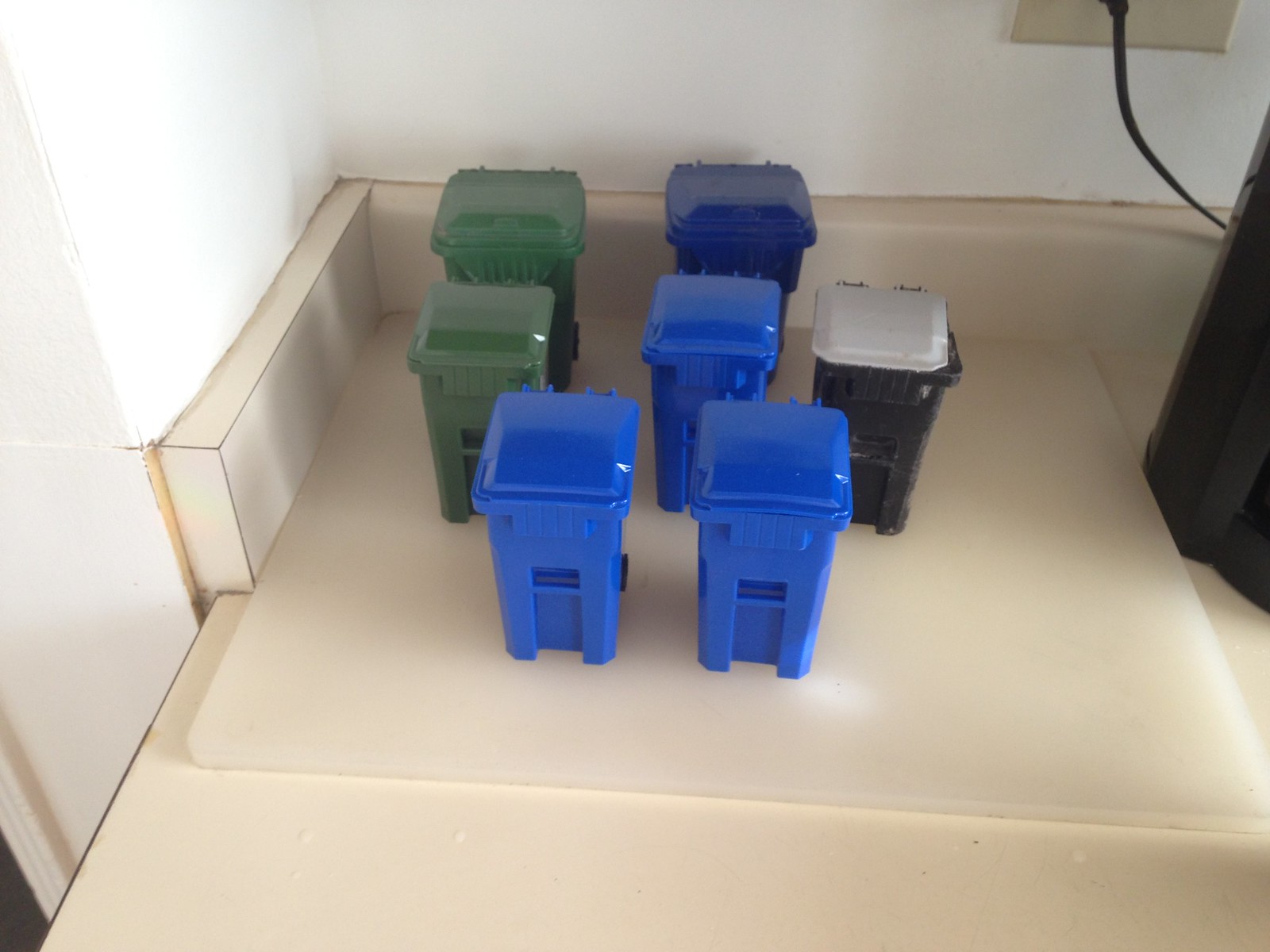This detailed photograph showcases seven miniature, colorful outdoor trash cans meticulously arranged on a white, smooth surface reminiscent of a countertop complete with a short backsplash. The cans, made of opaque plastic with slightly translucent, shiny lids, are organized in a structured manner—two green on the top left, three blue in the middle, and two at the bottom right, with one black can featuring a white lid positioned centrally to the right. Notably, a small electrical outlet visible on the upper right reinforces the miniature scale of these cans, reflecting a nuanced design typical of what you'd expect curbside on trash day, but in a much smaller form. The setup rests on a hazy white, possibly translucent rectangular board atop what appears to be a beige linoleum countertop. The counter is backed by a partial linoleum border that halts midway along the wall, which is stark white except for a black structure, likely a copier, on the far right. This intriguing setup possibly suggests a display or modeling arrangement at a trash can manufacturer.